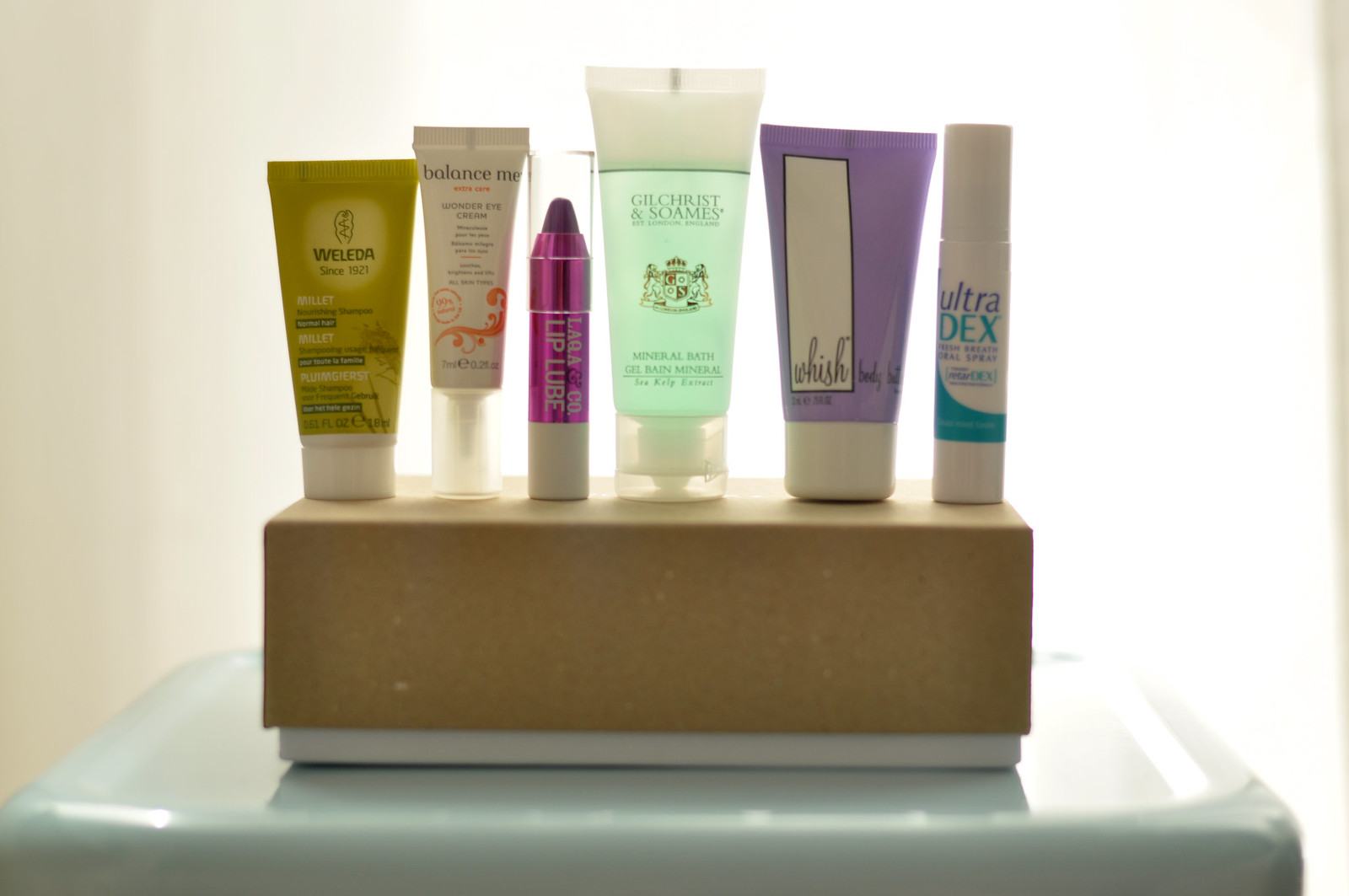This is a detailed horizontal photograph featuring a rectangular cardboard box with a brown top and a white bottom, the latter slightly peeking out. The side of the box is prominently displayed. On top of the box, six products are neatly arranged in a row:

1. The first item is a vertical bottle labeled "WELEDA" with a shape resembling an inverted trapezoid, wider at the top than the bottom.
2. Next to it is a white cylindrical product with a plastic cap. The word "balance" is written in lowercase black letters at the top.
3. The third product is a hot pink metallic lip crayon, featuring silver bands around the top and middle. The words "Lip Lube" are printed in all capital letters down the side, with the crayon tip visible and a plastic cap on top.
4. The fourth item is a white tube labeled "GILCHRIST & SOAMES" in all capital letters, with an emblem in the center and additional text below.
5. Adjacent to it is a light purple product. On its left side is a white vertical rectangle outlined in black, with the word "WHISH" written in black script inside. It has a white cap.
6. The final product is a round tube labeled "ultra" in lowercase blue letters, and "DEX" in turquoise capital letters. The predominantly white tube has a turquoise section extending horizontally across the left side.

The cardboard box is placed on a sleek, mint-green vinyl bench with a slight sheen. The bench is positioned against a cream-colored wall, and natural light illuminates the right side, creating a bright glow and lightly hitting the right side of the bench.